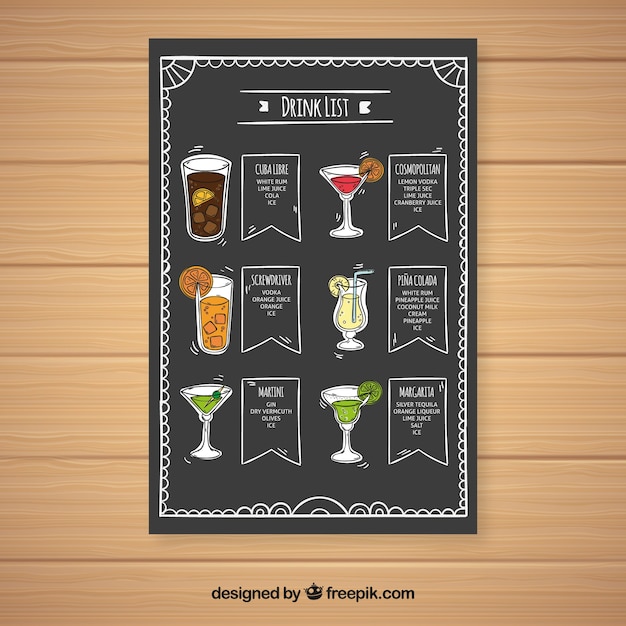The image features a drink list poster hanging on a wall that mimics the appearance of wood, but looks too pristine and is likely made of plastic. The poster itself consists of a black piece of paper with white, decorative frilly drawings in the corners and a title at the top in bold white lettering that reads "Drink List." The list showcases six different cocktails, each paired with a depiction of the drink and a detailed description of its ingredients. 

In the top left corner is the Cuba Libre, composed of white rum, lime juice, cola, and ice. Next to it is the Cosmopolitan, depicted with a red liquid in a martini glass, made from lemon vodka, triple sec, lime juice, cranberry juice, and ice. Below these are the Piña Colada, a light yellow drink made from white rum, pineapple juice, coconut milk, cream, pineapple, and ice, and the Margarita, containing silver tequila, orange liqueur, lime juice, salt, and ice. The list also includes the Screwdriver, made with vodka, orange juice, and ice, and the Martini, consisting of gin, dry vermouth, olives, and ice.

Each cocktail is illustrated with a graphic depiction, making the poster both informative and visually appealing. The Piña Colada and Cosmopolitan stand out visually, with the former appearing particularly refreshing.